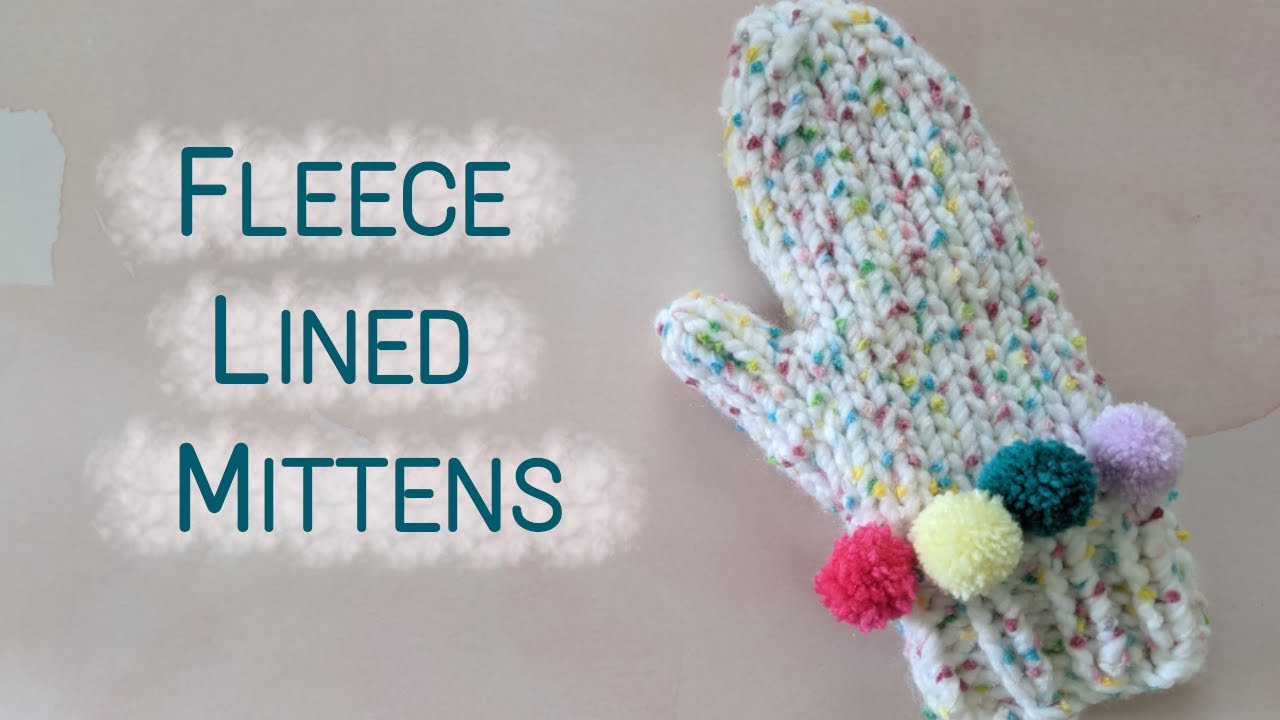The image features an advertisement showcasing a single fleece-lined mitten, positioned towards the right and slightly tilted to the left. This cozy mitten appears handmade, crafted from a white or off-white yarn adorned with speckles of vibrant colors including turquoise blue, bright yellow, burgundy red, and pink. Surrounding the wrist area are four pom-poms in shades of hot pink, light yellow, dark green, and lavender. The text on the left side of the image reads "fleece-lined mittens" in a dark teal or black font, set against a very light gray or foggy, snowy background. There is also a hint of light mocha color, as well as off-white areas adding to the soft, wintry aesthetic. The entire composition exudes a warm, festive feel, perfect for attracting attention to the cozy product.